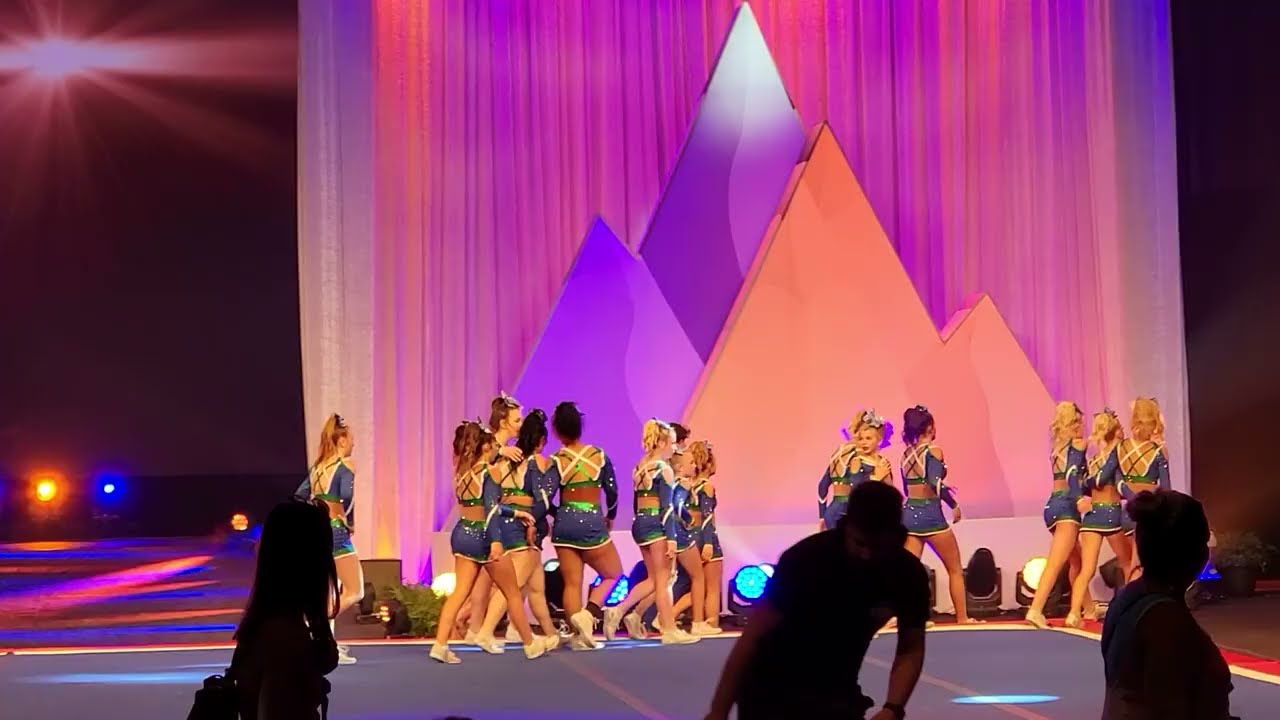The image captures a vibrant scene on a stage featuring a group of approximately 14 young girls, likely cheerleaders or dancers, dressed in sparkly blue mini skirt outfits with yellow trims and white sneakers. Their hair is styled in ponytails, often adorned with bows, and they appear to be wearing makeup. The stage backdrop includes colorful cardboard cutouts of mountains, with the tallest peak positioned centrally, painted white with a purple base. Smaller mountain cutouts flank this central peak, with the rightmost cutout in pinkish hues and the leftmost one in a purplish color, partially shadowed.

Behind the cutouts, purple and pink curtains drape down, complemented by a mix of stage lights – a bright white light from the top left, and blue and orange lights scattered across the lower left corner, near the bottom third of the stage. The lighting arrangement creates a dynamic play of colors, accentuating the scene.

In the foreground, three adults are seen in silhouette. On the left is a woman, followed by a man in the center seemingly rising from his seat while wearing a hat, and another woman on the right walking towards the left. The detailed setup indicates that the girls might be either preparing for or concluding a performance, as they appear to be milling about rather than standing in formation. The diversity among the girls is notable, with a mix of different ethnic backgrounds, creating an inclusive visual tableau.